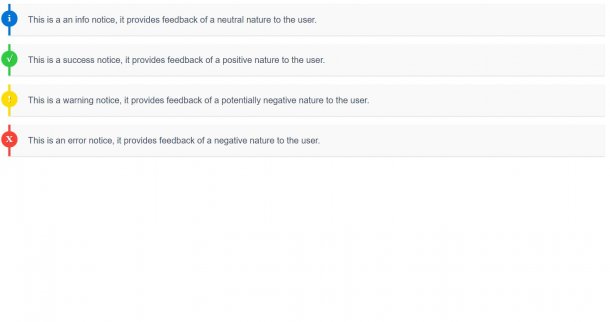The image features four rectangular light gray boxes, each containing a distinctive symbol and a descriptive message. 

1. **Top Box**: This box has a blue circle symbol on the left, with a vertical blue line at the top and bottom. Inside the circle is a lowercase "i." The accompanying text reads, "This is an Info notice. It provides feedback of a neutral nature to the user."

2. **Second Box**: Below the first, this box features a similar design but with a green circle and vertical green lines on the left. The text states, "This is a Success notice. It provides feedback of a positive nature to the user."

3. **Third Box**: The third box displays a yellow circle with vertical yellow lines on the left. The message reads, "This is a Warning notice. It provides feedback of a potentially negative nature to the user."

4. **Bottom Box**: The final box has a red circle with vertical red lines on the left, enclosing an "X" symbol. The text here says, "This is an Error notice. It provides feedback of a negative nature to the user."

The entire image has a white background, with thin strips of white space separating each of the gray boxes.